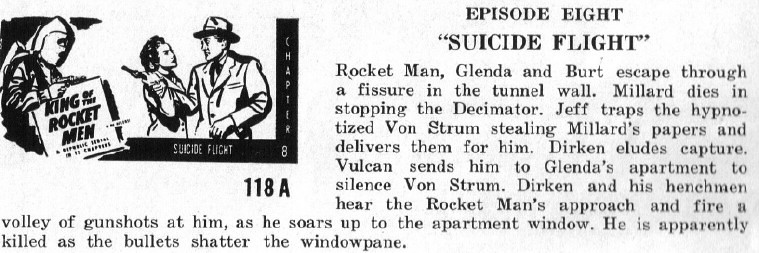The image appears to be a digitized clipping from an old newspaper, featuring both text and a photo. On the left side, the photo depicts three main figures: a man in a space outfit known as the "Rocketman," standing with his right hand extended and possibly holding a gun, facing right. To his right, there is a man dressed in a 1930s-style suit and hat, facing left, holding a gun that a woman next to him is attempting to take from his hand. Both the man in the suit and the woman have their right elbows bent, and the gun is pointing backward toward the Rocketman. 

The text next to the photo is titled "Episode 8, Suicide Flight," and it describes a dramatic sequence from a story. It reads, "Rocketman, Glinda, and Bert escape through a fissure in the tunnel wall. Miller dies stopping the decimator. Jeff traps the hypnotized Von Strom stealing Miller's papers and delivers them for him. Durkin eludes capture. Vulcan sends him to Glinda's apartment to silence Von Strom. Durkin and his henchmen hear the Rocketman's approach and fire a volley of gunshots at him as he soars up to the apartment window. He is apparently killed as the bullets shatter the window pane."

Adjacent to the photo, there is additional text and a black border indicating this is Chapter 8 of the story. The scene is from "King of the Rocket Men," with the serial episode explicitly noted as "Suicide Flight." Below the photo, the chapter number "118A" can be seen.